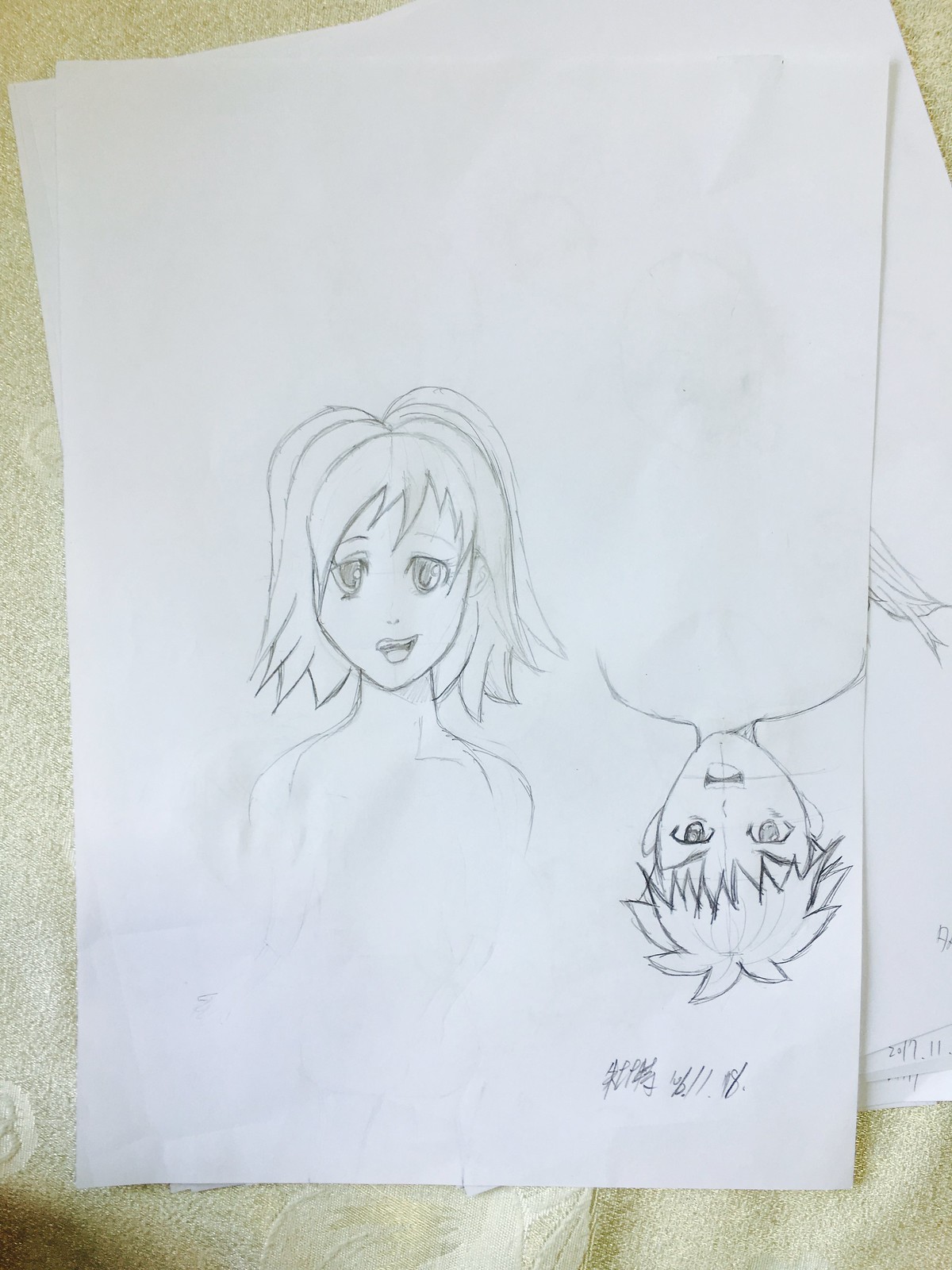This sketch features two children depicted in a stylized, somewhat anime-inspired manner. On the left, a girl with short, spiky hair that reaches her chin is smiling warmly. Her bangs frame a face characterized by unusually large eyes and a minimalistic nose. Opposite to her, an upside-down boy with equally spiky, short hair mirrors her exaggerated eye style and understated nose. He wears a plain shirt, though the focus remains predominantly on their faces. Both characters exude a whimsical and slightly surreal charm. Above the boy's head, there is a small doodle, possibly serving as the artist's signature.